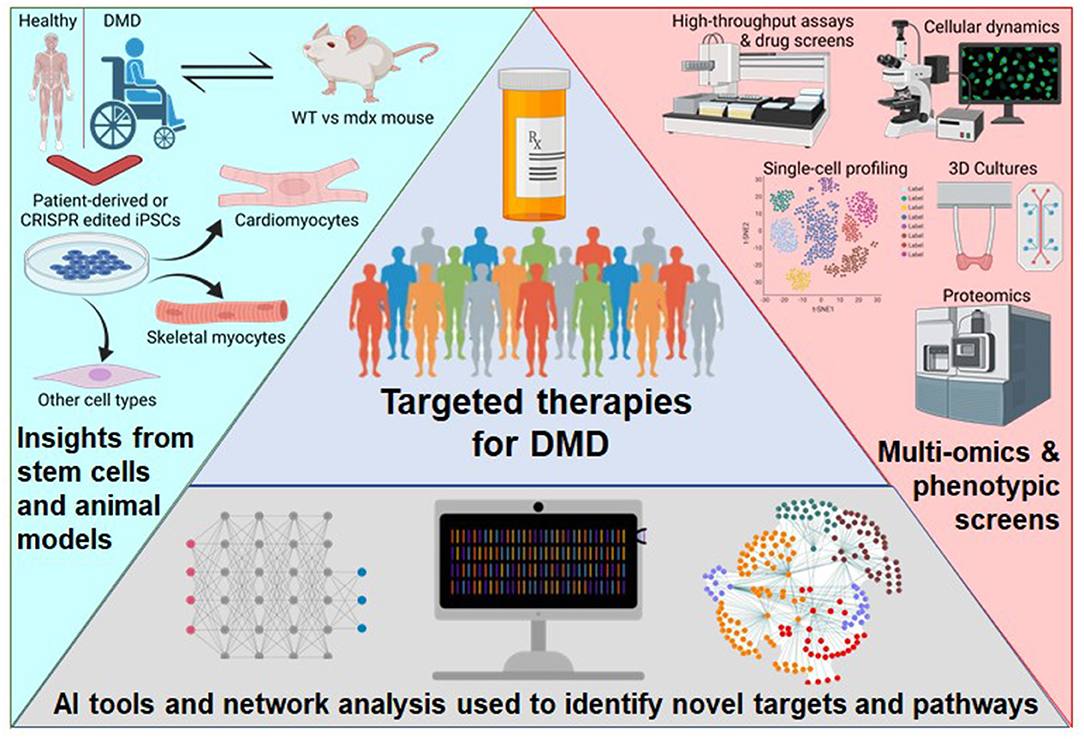The image is a detailed and segmented diagram, primarily focused on various aspects of medical research and treatments for Duchenne Muscular Dystrophy (DMD). The diagram is structured as a rectangle composed of different triangular sections.

The central portion of the image highlights the text "Targeted Therapies for DMD," surrounded by multicolored cartoon-like human figures, symbolizing diverse patient demographics. Above this central text is an icon of an RX bottle, emphasizing medication.

To the left is a segment with a light blue background. This area depicts a healthy human figure and a DMD patient in a wheelchair, each labeled accordingly. There are arrows pointing to a white mouse labeled "WT versus MDX mouse," illustrating animal models used in research. Below this, a Petri dish labeled "Patient Derived or CRISPR Edited iPSCs" shows different cell types—cardiomyocytes, skeletal myocytes, and others. This section is titled "Insights from Stem Cells and Animal Models."

The right side, set against a pink background, showcases various lab equipment and methodologies under headings such as "High Throughput Assays and Drug Screens," "Cellular Dynamics," "Single Cell Profiling," "3D Cultures," and "Proteomics." At the bottom, it mentions "Multiomics and Phenotypic Screens."

The bottom section of the central area, with a gray background, states "AI Tools and Network Analysis Used to Identify Novel Targets and Pathways." It features a computer screen accompanied by graphs and a network web, symbolizing the integration of artificial intelligence in medical research.

Overall, the diagram provides a comprehensive overview of the multi-faceted approach to DMD treatment and research, incorporating elements from stem cells and animal models to advanced AI tools and various lab techniques.